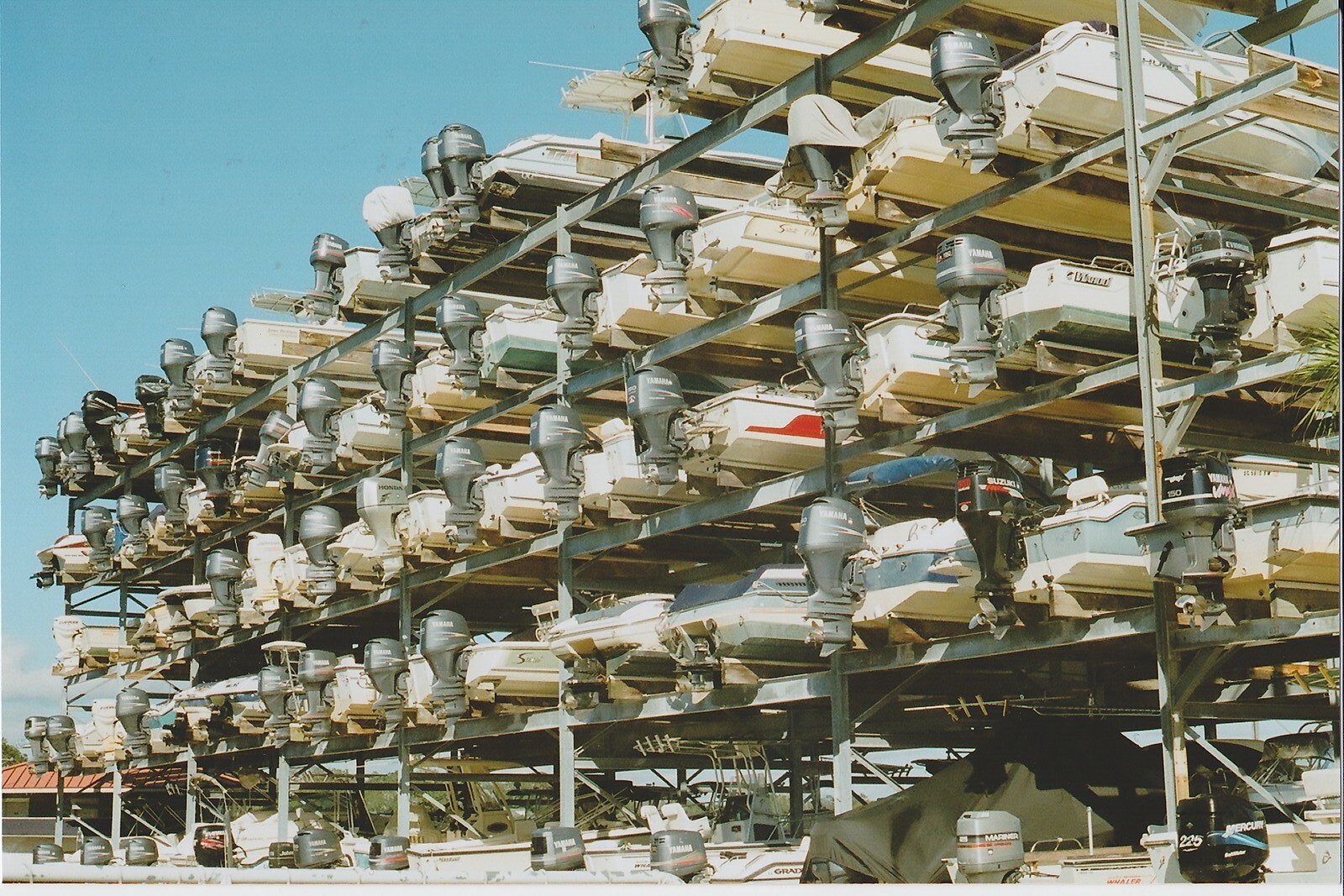The photograph captures a sprawling, open-air boat storage facility at a marina. The massive, steel-framed structure stretches from the bottom right to the top left of the image, narrowing as it recedes into the distance. The facility holds rows upon rows of boats, packed tightly like sardines, with each row accommodating around 10 to 16 boats across its five visible levels. These boat racks, resembling tall scaffolding, house at least 80 boats in various sizes and colors, though many are white or cream-colored. Some boats feature single or double outboard engines. Beneath the towering racks is additional parking for more boats. The bottom-left corner of the image includes the clay-colored, terracotta roof of a low building, likely the marina offices. The scene is backed by a clear blue sky, visible primarily in the upper left-hand portion of the photograph, adding a serene backdrop to the bustling storage area. The entire structure appears to be anchored into a cement base, possibly extending underwater, embodying an efficient, albeit densely packed, dry dock storage solution.